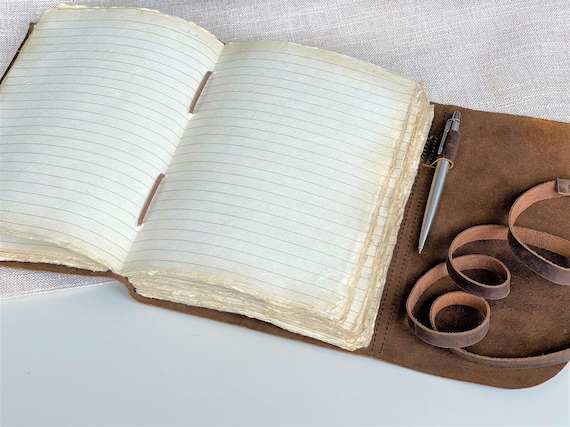The photograph captures an old-fashioned, open diary or journal with jagged, raw edges, adding to its vintage appeal. The pages are blank and lined, showing signs of wear, giving it a faded, well-used look. At the center of the notebook, two thin, cord-like pieces of string, possibly brown leather, are visible, likely contributing to its binding. This notebook is nestled within an open brown leather portfolio, which has a coiled leather strap. Inside the portfolio, there is a silver pen secured neatly in a dedicated pen slot. The entire setup is partially laid on a beige fabric atop a gray-beige table, possibly a white table with a tablecloth, enhancing the rustic and aged feel of the scene.